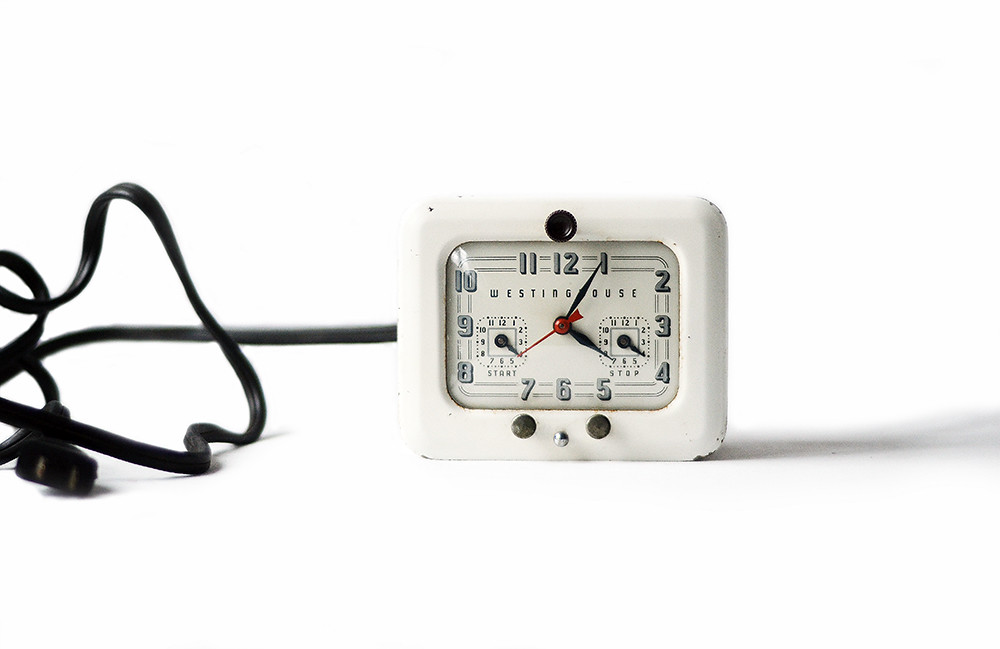The image showcases a small, vintage, square-shaped white alarm clock branded "Westinghouse". The clock's design is notably old-fashioned, with a rectangular clock face that's segmented into four groups of numbers: 11, 12, and 1 at the top; 2, 3, and 4 on the right; 7, 6, and 5 at the bottom; and 10, 9, and 8 on the left. The clock hands consist of a red second hand and black hour and minute hands, with the minute hand positioned near 1 and the hour hand between 4 and 5. The face includes two smaller dials—likely auxiliary time or measurement displays—labeled with unclear words that might be "store" on the left and "beep" on the right, each with a single hand and numbered 1 to 12. The background is plain white, allowing a shadow to extend to the right of the clock. A long black power cord emerges from the back, curving left and ending in a visible plug. The clock features additional controls: a black button on top, two black buttons and a small silver knob on the bottom front.